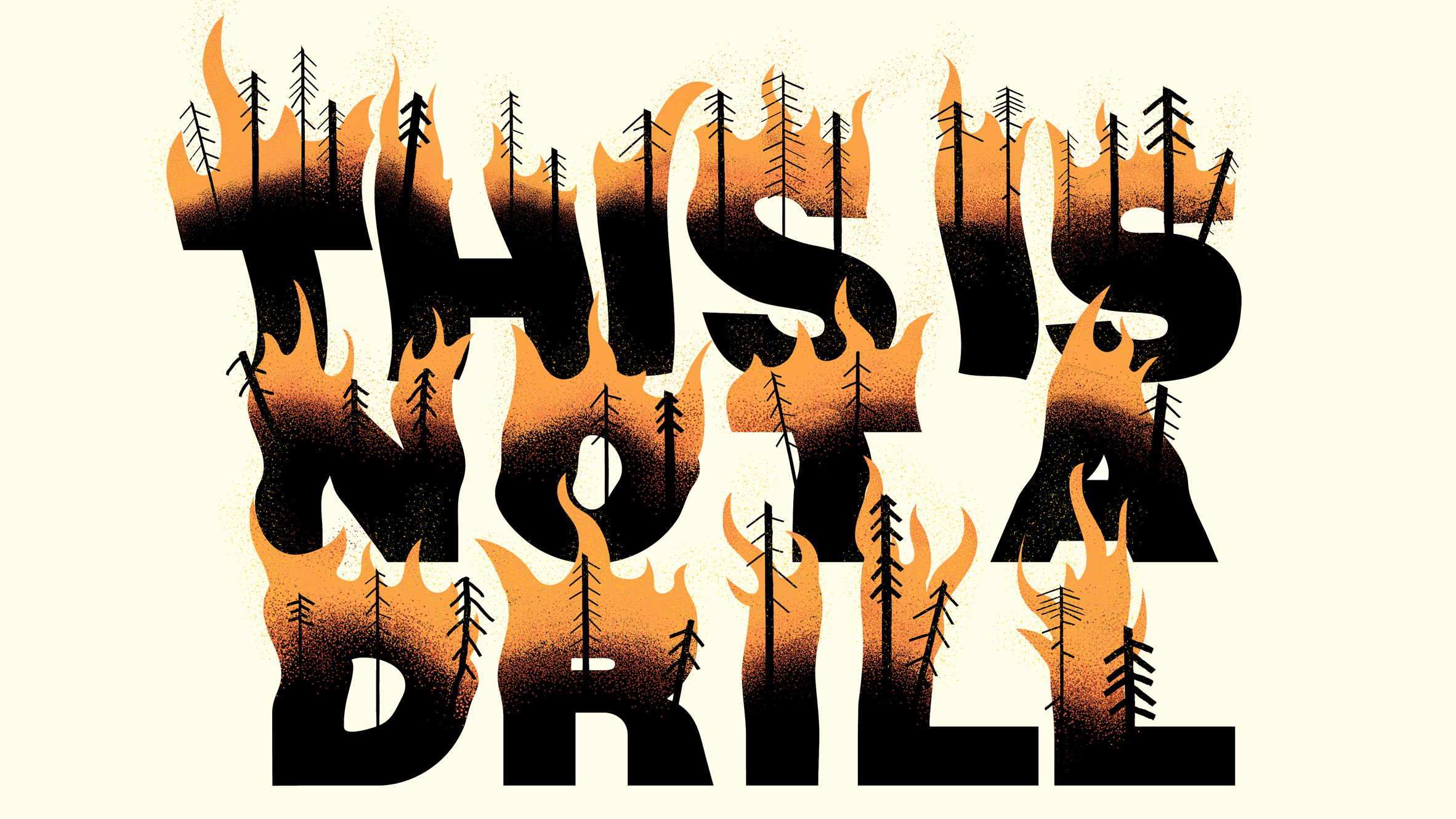The image is a striking illustration resembling a logo or signage with the text "This is not a drill." The text is rendered in thick black letters, arranged in a stacked format: "T-H-I-S" on the first line, "I-S" on the second, "N-O-T" on the third, "A" on the fourth, and "D-R-I-L-L" on the fifth. Each letter transforms vividly from a solid black base into a dramatic depiction of a forest fire. The lower portion of each letter maintains a clear, bold black form, which gradually morphs upwards into silhouettes of bare trees. These trees then transition into vivid flames that engulf the upper parts of the letters, giving the appearance that the lettering itself is burning. This blazing effect creates a sense of urgency and realism, simulating an actual forest fire. The background is a neutral beige, enhancing the impact of the black and fiery elements of the design, which may be intended for a t-shirt or as a warning sign related to forestry. The dynamic visual suggests a powerful warning, capturing attention with its fiery transformation from the base of each letter to the top.